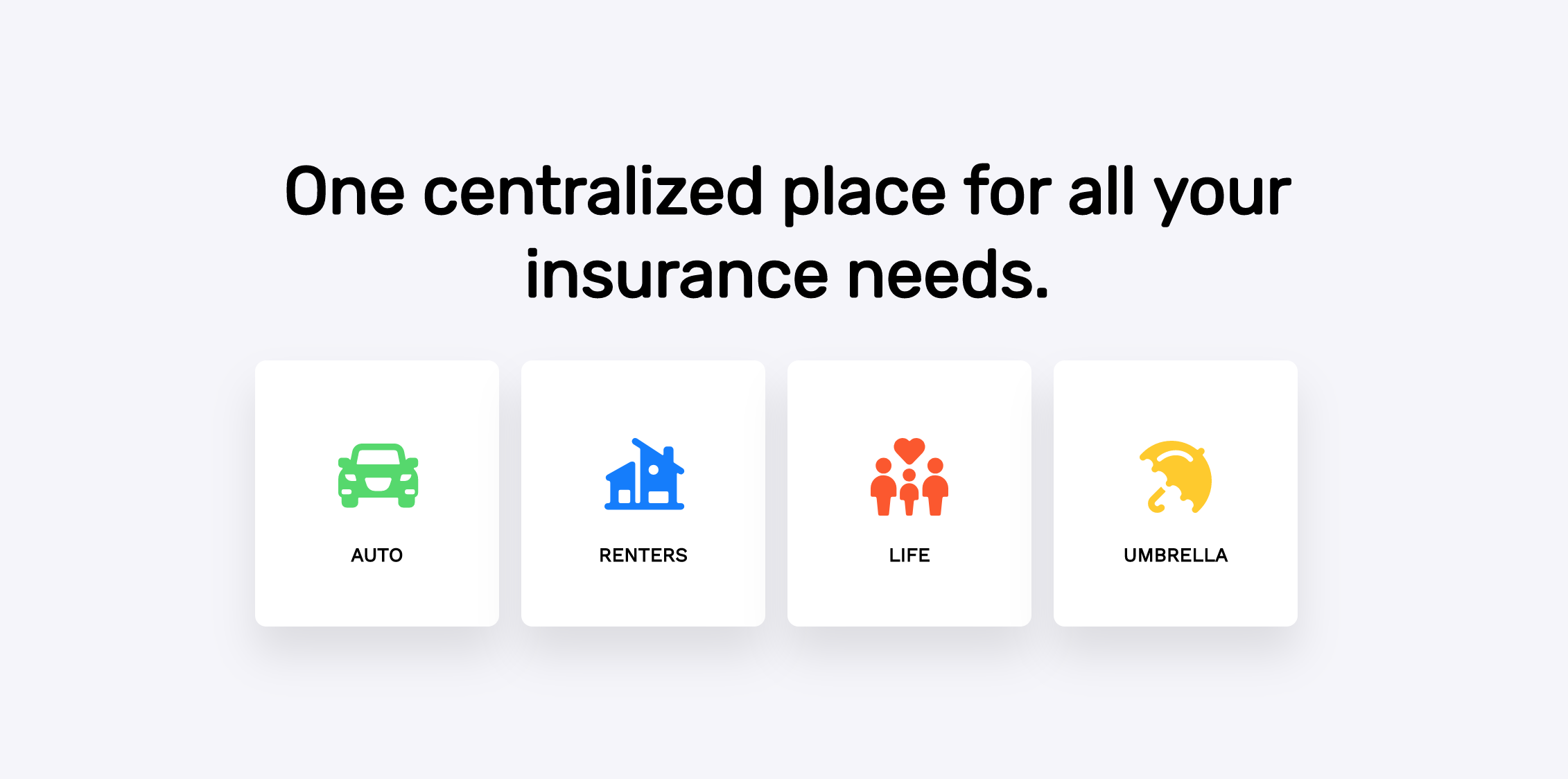A panoramic image with a faint blue background serves as the backdrop for an insurance advertisement. Dominating the upper portion of the image, large black text reads, "One centralized place for all your," with "insurance needs" centered directly below on a separate line. Positioned just below the midpoint of the image are four distinct white squares, each containing an icon related to different types of insurance. From left to right:

1. The first square features a green car icon facing forward, accompanied by the word "AUTO" in black, all-capital letters beneath it.
2. The second square displays an icon of two blue houses, with the word "RENTERS" in black, all-capital letters situated below.
3. The third square depicts an icon of three figures—a man, a woman, and a child—centered under a heart. The icon is in orange, and the word "LIFE" appears in black, all-capital letters below it.
4. The fourth square contains a yellow umbrella icon, with the word "UMBRELLA" in black, all-capital letters underneath.

Overall, the image presents a clear and organized visual prompt, emphasizing the availability of various insurance options in a straightforward and minimalistic manner.